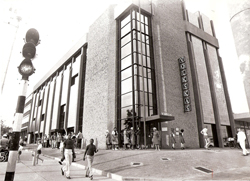This black-and-white photograph showcases a bustling city scene, centering on a towering building adorned with numerous architectural details, including many tall windows and window panes. The structure, likely a department store or institution, rises majestically towards the top of the image. The front corner features a striking glass facade, flanked by concrete walls. A stone canopy juts out from the entrance. The scene is alive with activity: numerous people are milling about, with many entering and exiting the building, and others walking along the clean concrete sidewalks. Prominently featured are two individuals in white pants and dark tops. The left side of the frame includes an old-fashioned, striped lamppost, hinting at the photograph's historical context. Despite some text visible on the building, its letters remain unreadable. The surroundings include a large cement apron area and a stoplight in the foreground, adding to the urban atmosphere.